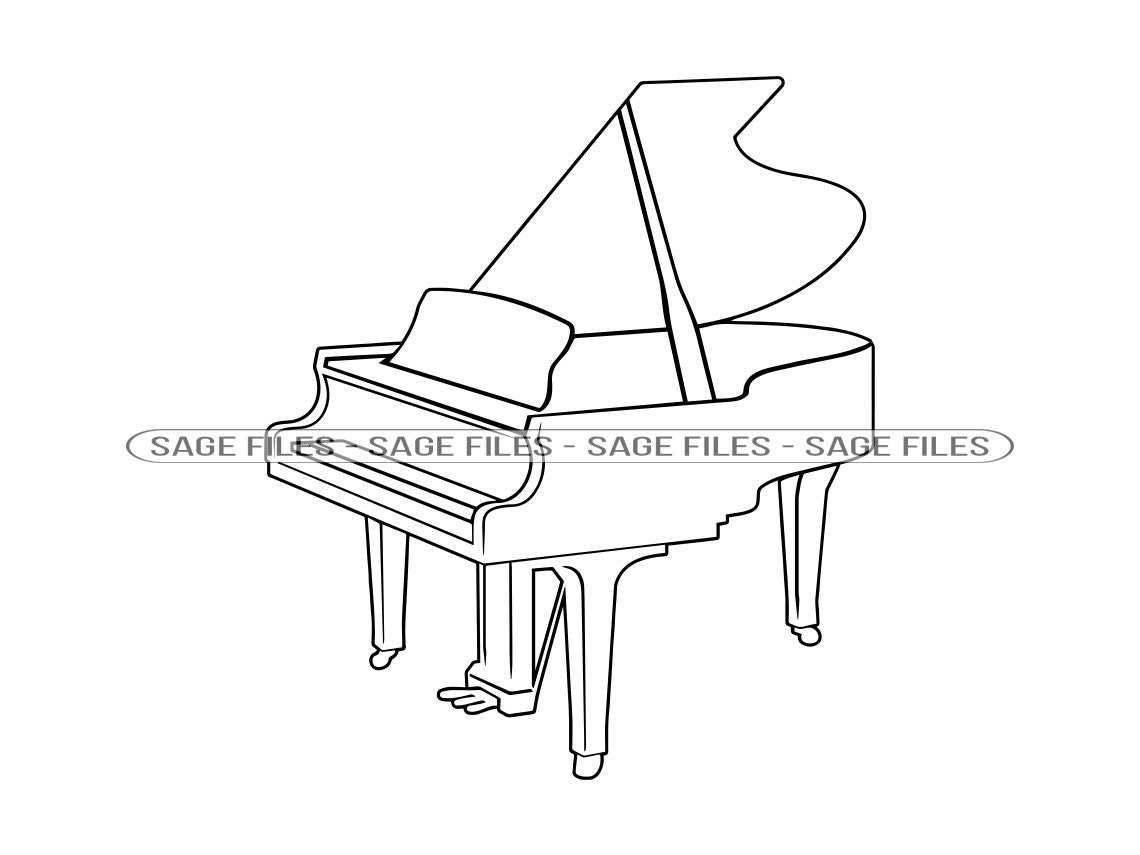This image depicts a minimalistic, black and white, pencil-drawn outline of a grand piano, with the top lid propped open, exposing the strings and soundboard. A watermark reading "Sage Files" appears four times in an oval pattern across the center of the image. The piano stands alone against a stark white background, with no additional elements such as a bench or sheet music. The keys appear to be covered, and the detailed illustration includes the legs and feet of the piano, as well as three foot pedals at the bottom. This clean and simple rendering focuses on the essential features of a grand piano, emphasizing its elegant form.